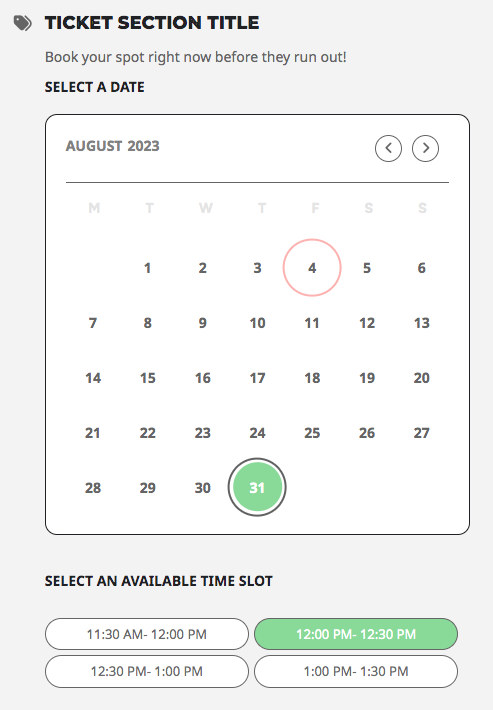This image is a cropped screenshot from a website, focusing on a pop-up selection window with a grey background and black text. The window is titled "Ticket Section Title". In smaller grey text beneath the title, it says, "Book your spot right now before they run out."

Below this, a bold, capitalized instruction reads "SELECT A DATE", accompanying a calendar for the month of August 2023. Within the calendar, the date Friday, August 4th is marked with a red circle, while Thursday, August 31st is highlighted with a green circle.

At the bottom of the window, there is an option to select an available time slot. Four selectable times are listed: 

- 11:30 AM to 12:00 PM
- 12:00 PM to 12:30 PM (this slot is highlighted in green, indicating it has been selected)
- 12:30 PM to 1:00 PM
- 1:00 PM to 1:30 PM